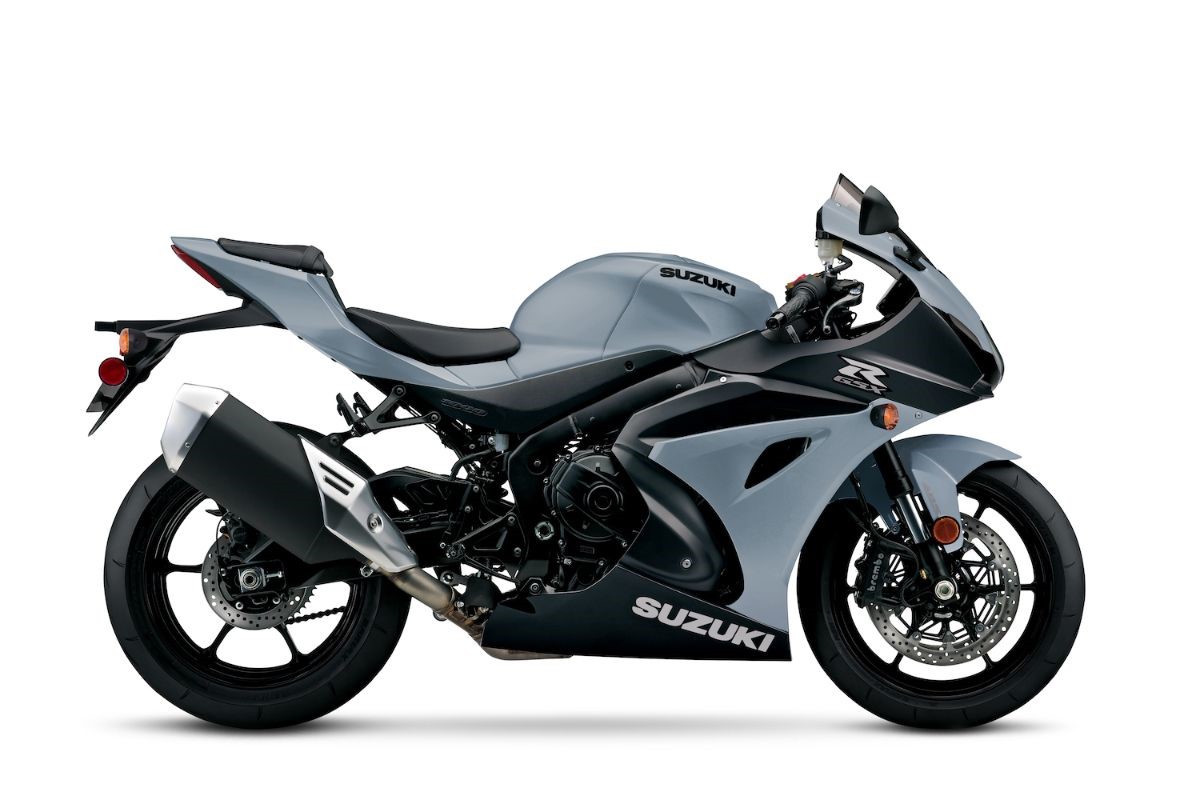This image features a modern, high-tech Suzuki motorcycle predominantly in black with various grey and blue accents. The name "Suzuki" appears in black on the gas tank, and in white on the base of the bike. The motorcycle sports a "GSX" logo with an "R" below the grey windshield. The design emphasizes a black windscreen with rear-view mirrors and a handlebar equipped with brakes and controls. The seat and body are primarily grey, with some baby blue-like steel elements adding a sleek touch.

The front of the motorcycle, situated to the right, highlights a light grey fender with black tires featuring spokes extending from rims. The sophisticated suspension system includes visible shocks and a chain drive connected to the sprocket, with disc brakes for efficient stopping power. The engine appears air-cooled and is partially shielded by a black protective plate. 

The exhaust system showcases a chrome-tipped muffler with varying sections of chrome and silver piping. The lighting fixtures include orange and red glass for the rear and brake lights, with a detached section at the rear for blinkers mounted on a small stick-like extension. The overall design suggests that the rider would adopt a forward-leaning posture, typical of many Japanese sport bikes.